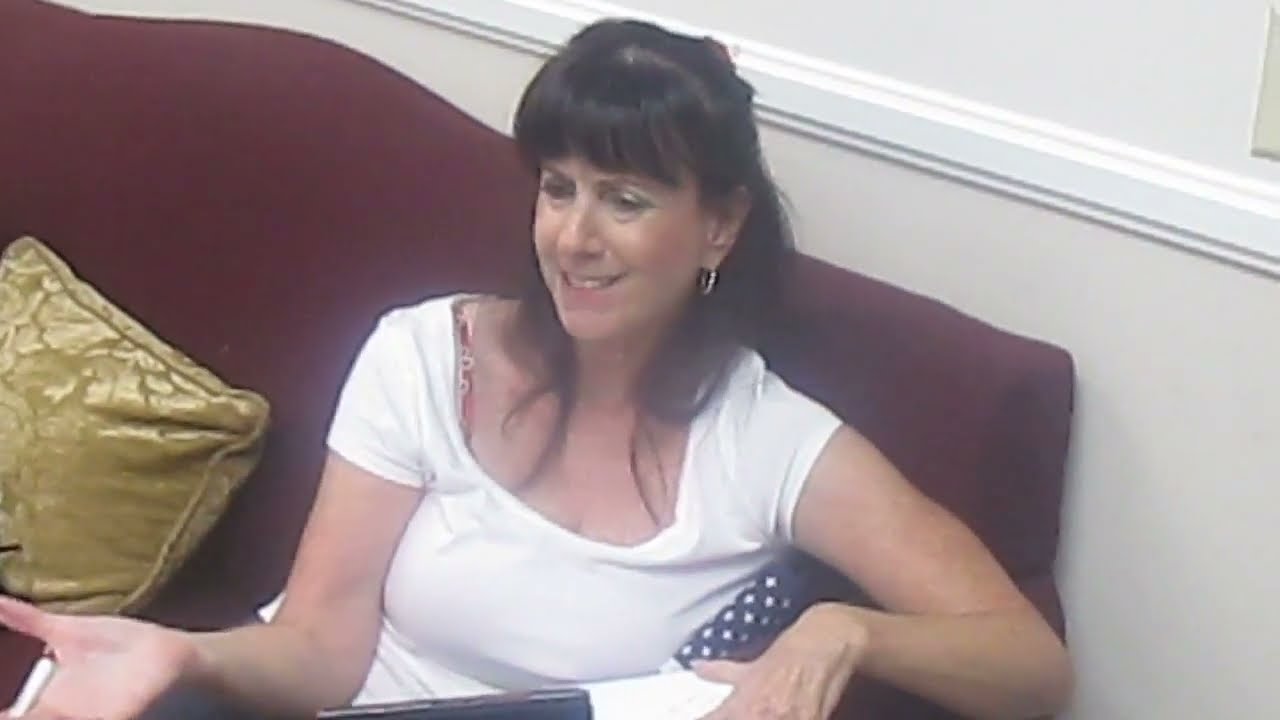In this compelling image, we see a woman deeply engaged in a conversation, her expression a mix of grimacing and making a point. She is seated on a luxurious burgundy velvet couch adorned with two pillows: a vibrant gold one and a black polka dot one for support. The woman is dressed in a white short-sleeved top that slips slightly off her shoulder, revealing a bra strap. Her long black hair cascades around her face, framing her expressive features, and she wears hoop earrings that add a touch of elegance. Her hand is extended with the palm up, as if emphasizing a point, while beside her, an American flag with its blue field and white stars is draped over the wooden armrest of the couch. The background is a pristine white wall with intricate molding, completing the intimate setting of the room.